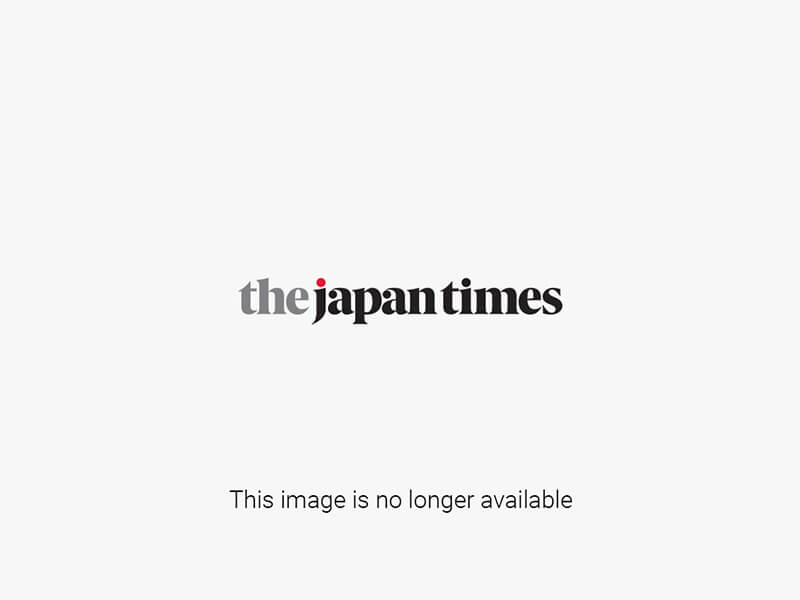The image features an Asian male figure skater dressed entirely in black, performing on an ice rink. He dons long black pants and a short-sleeve black athletic shirt with gray patches on both shoulders. His black skates are distinguished by small, yellow writing on the heel of the left skate. His striking appearance is accentuated by his spiky black hair and the various accessories he wears—black bead bracelets on his right wrist, a bracelet with predominantly white beads and a few black beads on his left wrist, and a necklace on a black thong around his neck. His t-shirt may also feature small, unreadable white text on a breast pocket. The skater is captured in a dynamic pose that suggests he is in the middle of a turn or spin, with his right hand extended to the side and his left hand positioned behind him for balance. The background of the image is minimalistic, showcasing a smooth, white ice surface and a featureless white wall with a yellow border at the bottom.